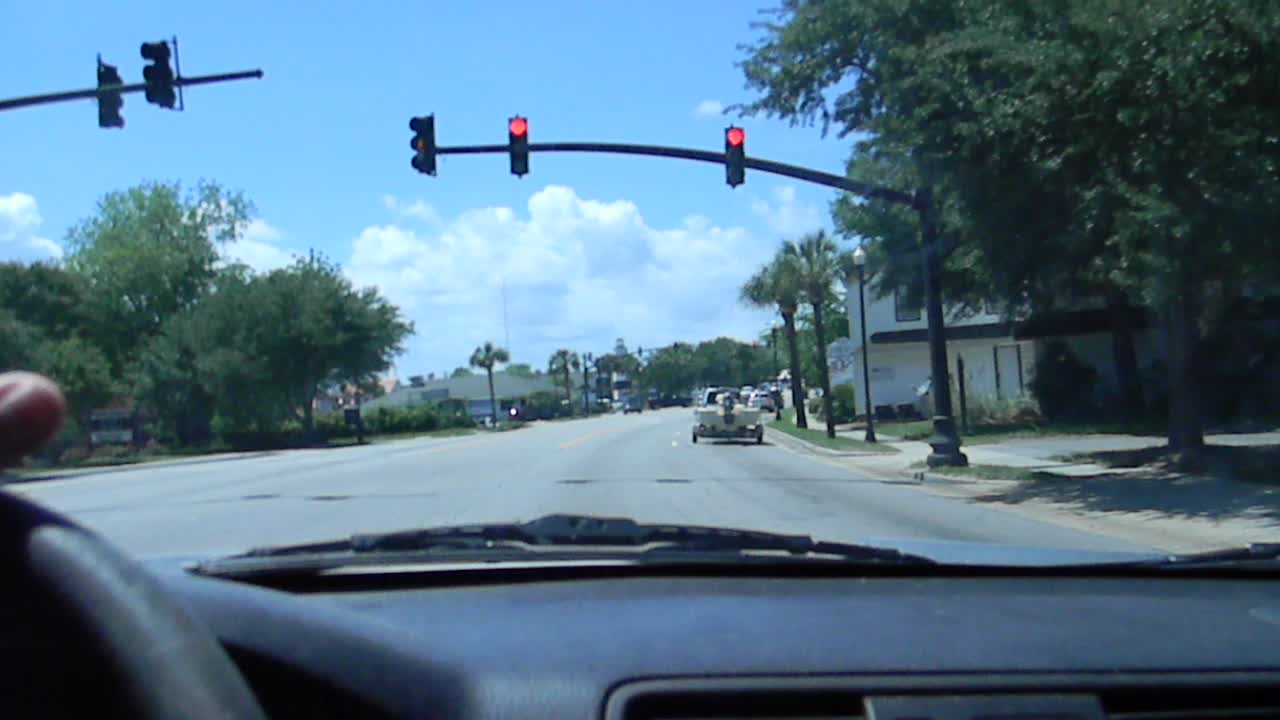The image captures the driver's perspective from inside a car, halted at a red traffic light at an intersection. About 30% of the steering wheel is visible in the lower left corner, along with the driver's thumb, nail pointing towards the camera. The dashboard is in view, as are the windshield wipers seen through the clear windshield. Ahead lies the road, with two prominent red traffic lights mounted on a pole emerging from the ground on the right. This pole stands adjacent to a lush, green tree, and several pine trees are discernible below the traffic lights. In the right lane, a dark-colored boat is visible, being towed by a pickup truck. The background features a mix of buildings and additional trees. Above, the sky is a brilliant blue, adorned with puffy white clouds, complementing the serene scene.